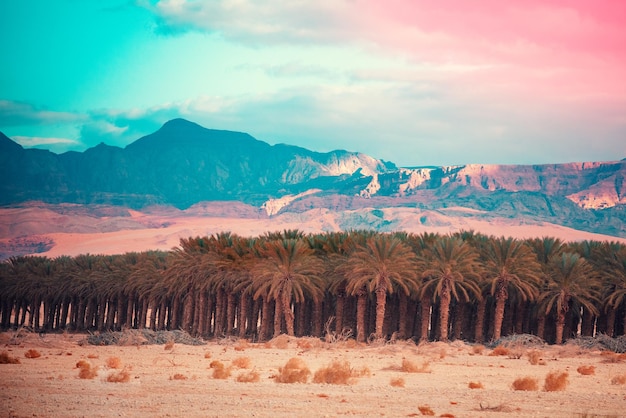This is a horizontal photograph capturing a tropical island oasis amidst a desert-like setting. The viewer is positioned at a distance from a dense tree line of palm trees, which predominantly appear brown due to a muted, possible filter effect. Just before this tree line lies a sandy beach scattered with brown vegetation or tumbleweeds. The background reveals a stunning mountain range with hues transitioning from blue to snow-capped white as they ascend. Above the mountains, the sky is uniquely tinted, with the left side displaying a turquoise blue reflecting down on the highest peak, and the right side showcasing pinkish-red tones through a cloud-heavy sky, giving the scene an ethereal appearance. The overall color palette of the image is subdued, suggesting the use of a filter or capture on a hazy day, contributing to an almost surreal depiction of this deserted oasis landscape.